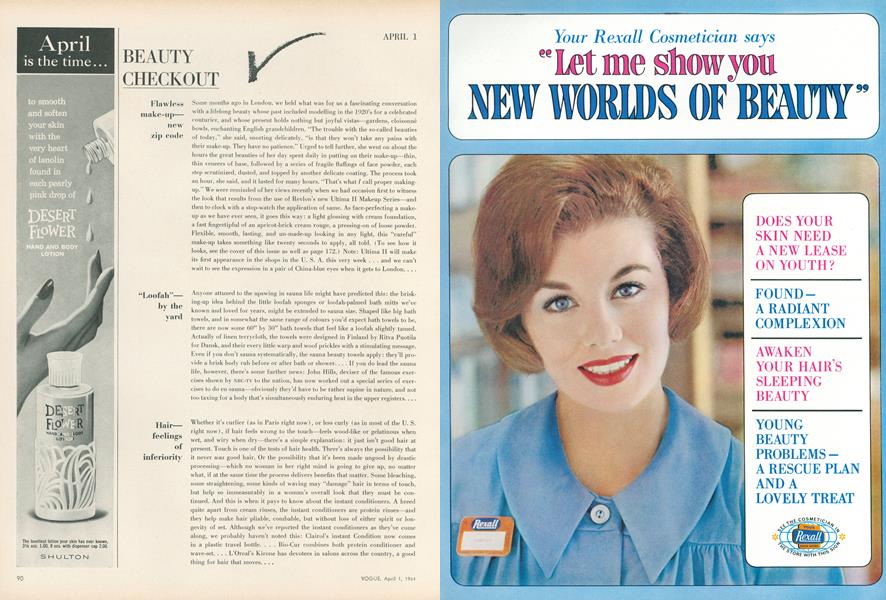This image captures a vibrant and nostalgic two-page spread from a vintage Vogue magazine, dated April 1st, 1964. The left page, set against a tan background, features a black-and-white vertical ad column titled "Beauty Checkout," showcasing an image of a hand with lotion being poured on it, accompanied by a bottle labeled “Desert Flower” hand and body lotion. The ad text begins with "April is the time to smooth and soften your skin with the very heart of a pink drop desert flower." The right page, contrasted in a light blue hue, is headlined by "Your Rexall Cosmetician says, Let me show you new worlds of beauty." Dominating this page is a colored photograph of a woman with a 1960s-style pixie haircut, bright red lipstick, and a blue top with a large pointed collar and pleats. She smiles warmly at the viewer while wearing a Rexall name tag. The page is interspersed with various snippets of text including, "Does your skin need a new lease on youth?" and other beauty tips. This spread vividly captures the essence of 1960s beauty and fashion advertising.